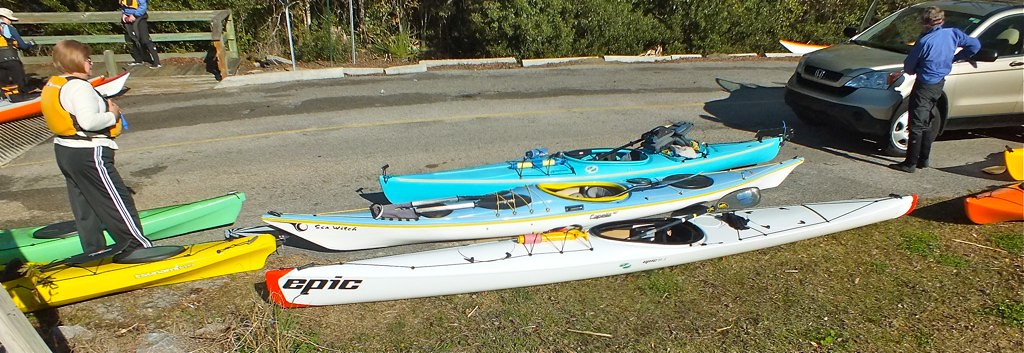This photograph captures a dynamic scene centered around a group of kayaks and people, likely preparing for a kayaking trip or returning from one. Central to the image are three prominently displayed kayaks: two in blue and white hues, and a distinct white kayak accented with red, bearing the word "Epic" on its left side. Adjacent to these main kayaks, on the left, stands a middle-aged white woman dressed in black pants with a white stripe, a white long-sleeve shirt, and a yellow and black life vest. Nearby her are two smaller kayaks, one lime green and the other yellow. To the right, parts of two other kayaks—one orange and one yellow—are visible.

A man dressed in black pants and a black shirt stands near a silver, small SUV, likely a Honda, which is parked close to the edge of an asphalt road that might lead to a park or parking lot. The scene includes a total of eight kayaks scattered around, some stacked and others lying individually. In the background, we see a wooden walkway or deck with people standing on it, including some wearing life jackets, suggesting they are also involved in kayaking.

The setting is under a bright, sunny sky characteristic of a summer day, casting light on the browning grass and the general dry condition of the area. Further adding to the sense of activity, the background reveals a two-lane street lined with trees at their bases, reinforcing the likely proximity to a natural park or recreational area.